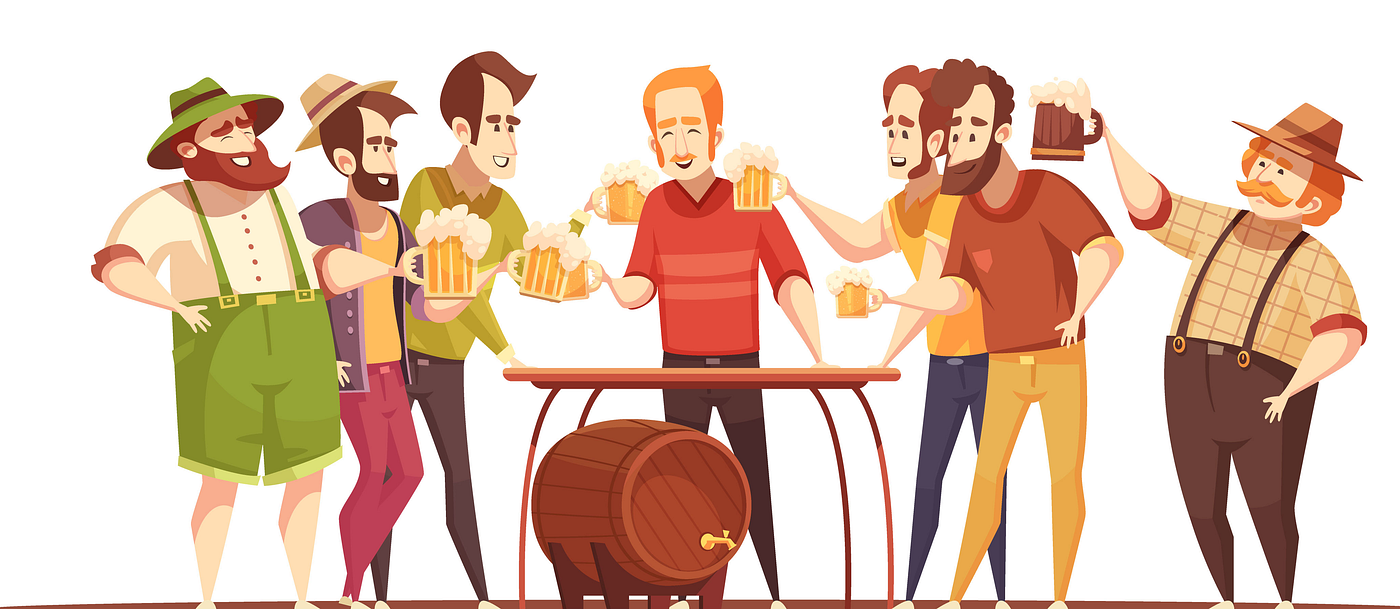A vibrant cartoon depicts a lively scene of seven men surrounding a small table with a beer keg underneath. Each man holds a foaming beer mug filled with amber-colored beer. The men, dressed in an eclectic mix of attire, ranging from traditional lederhosen and shorts with suspenders to t-shirts, long pants, and even a jean jacket with purple pants, create a colorful and dynamic tableau. Notably, some wear hats, contributing to their varied appearances. At the center of the scene stands a red-haired man in a red shirt, who seems to be the focal point, drawing the attention and raised glasses of the surrounding men. The first man is notably jovial, wearing lime green shorts and overalls paired with a tan shirt and a green hat. The overall mood is cheerful, with everyone appearing happy and laughing, contributing to an atmosphere of camaraderie and celebration.